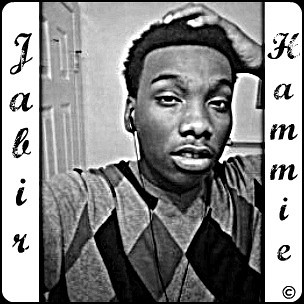The image features a black-and-white photograph with a central focus on an African American male, possibly intended as an album cover or a social media post. The man, located in the center of the image, is depicted with short, thick black hair and is wearing headphones. His hand rests on the top of his head, and he dons a shirt adorned with a diamond or checkered pattern. The backdrop reveals a closed door, adding to the setting's intimate, likely personal space. Vertical cursive letters spell "JABIR" on the far left and "KAMMIE" on the far right, with a copyright logo nearby, suggesting that these names may be of significance to the image, possibly the individual's full name. The overall monochromatic theme blends different shades of black, white, and gray, emphasizing a stylistic and personal atmosphere.